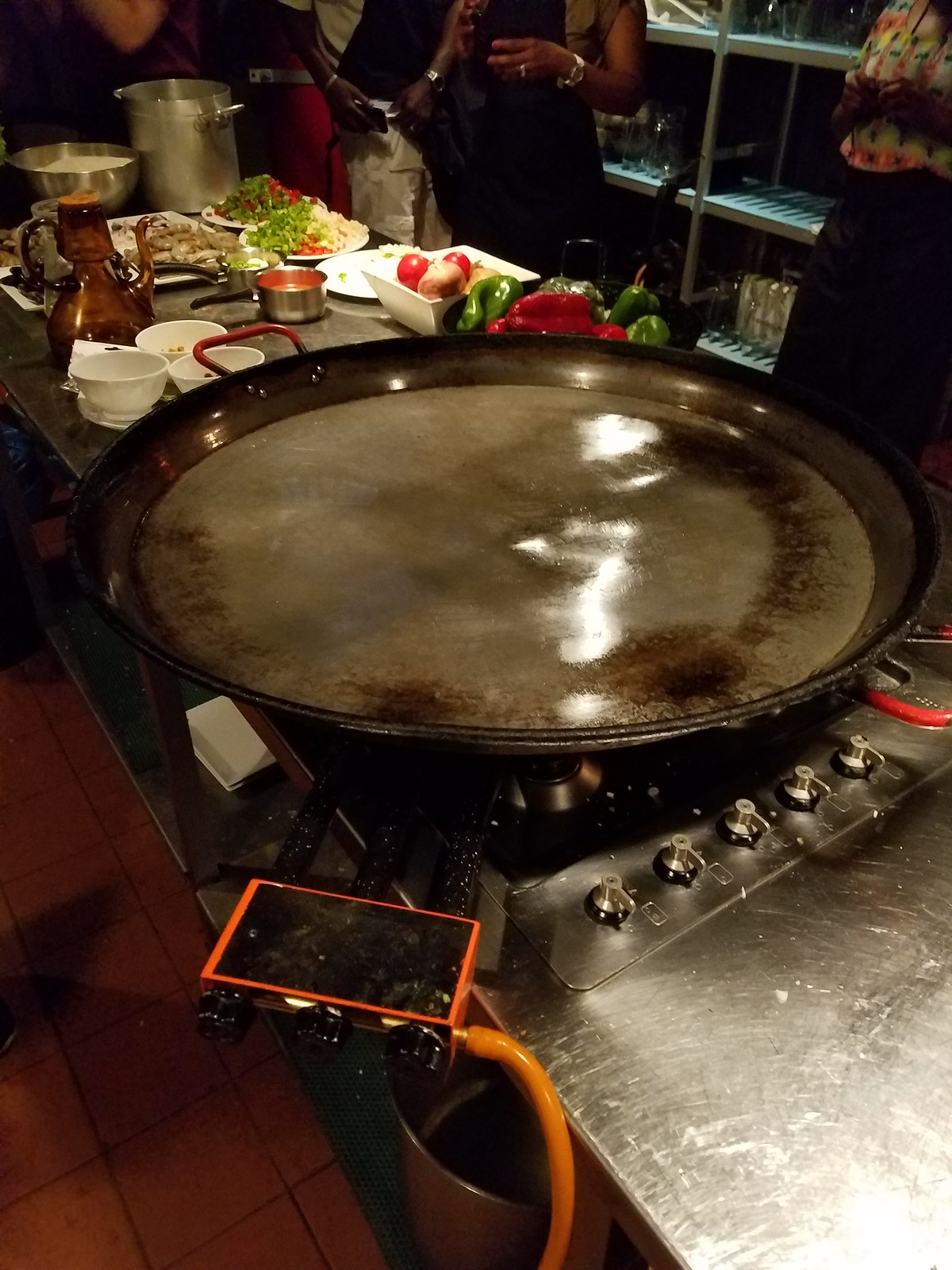In this image, we see a bustling cooking station crowded with activity. Several people, some wearing aprons and others in more formal attire, stand around a large, round griddle top that spans across four stove burners. This substantial piece of equipment is designed for high-heat cooking, evident from the array of control knobs and buttons along its side. The station is laden with various prepped ingredients, including bowls of vibrant red and green peppers, tomatoes, and other vegetables, as well as proteins. There are also ramekins, plates, and trays filled with different items, and a large silver pot and skillet are part of the setup. A pitcher, possibly containing oil, sits nearby, ready for use. This scene captures the anticipation of an intense and dynamic cooking session.